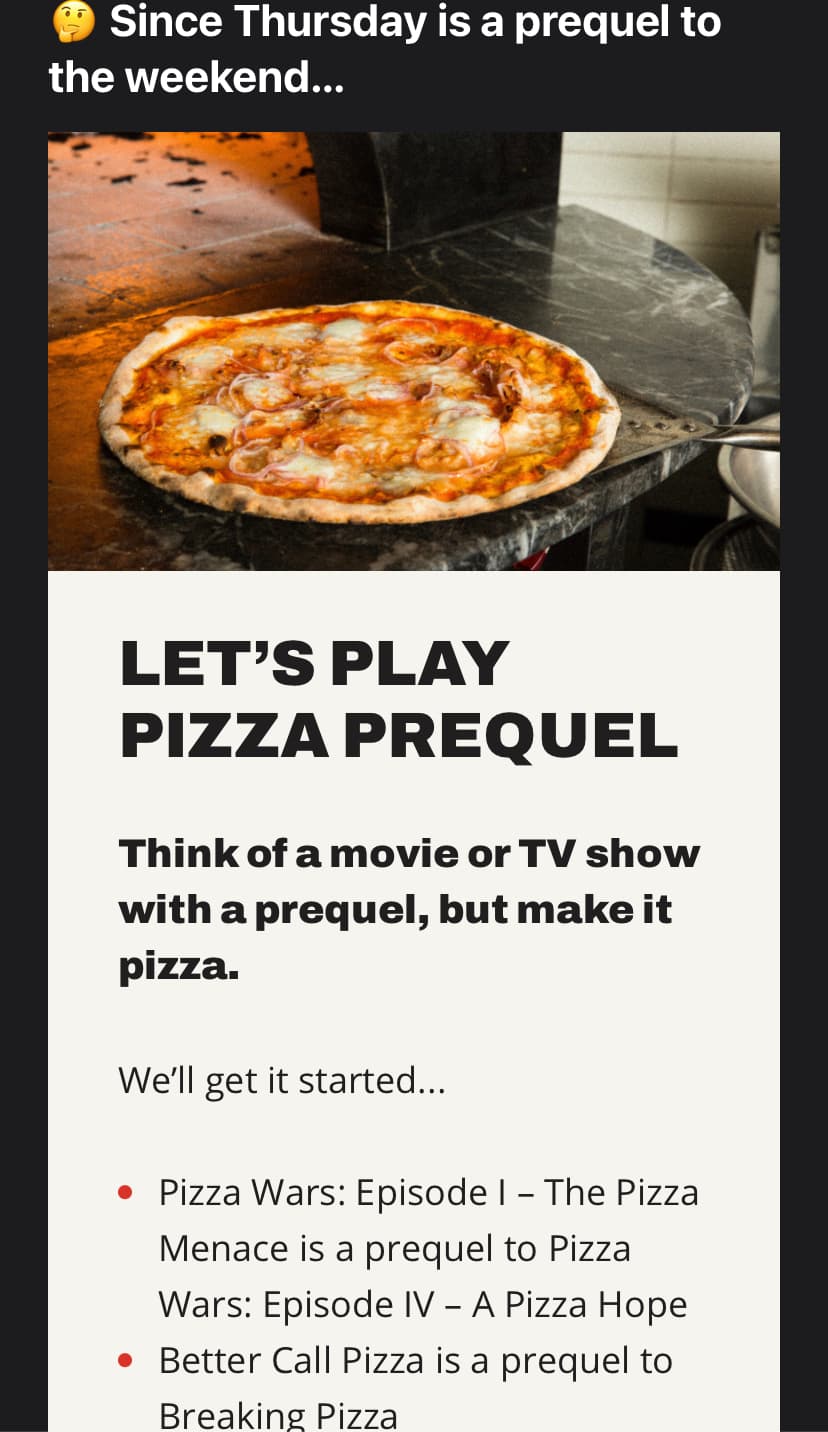Vertical flyer advertising a themed event centered around pizza prequels. The flyer features a black border and, at the top, an emoji with a puzzled expression, accompanied by text in white: "Since Thursday is a prequel to the weekend..."

Below, there is an image of a stovetop pizza poised to enter a large oven. Further down, the background turns white with prominent, bold letters proclaiming: "Let's Play Pizza Prequel". In smaller bold letters, it adds: "Think of a movie or TV show with a prequel, but make it pizza."

In regular, smaller font, it continues: "We’ll get it started..."

Two red bullet points follow:
1. "Pizza Wars Episode I: The Pizza Menace" is a prequel to "Pizza Wars Episode IV: A Pizza Hope".
2. "Better Call Pizza" is a prequel to "Breaking Pizza".